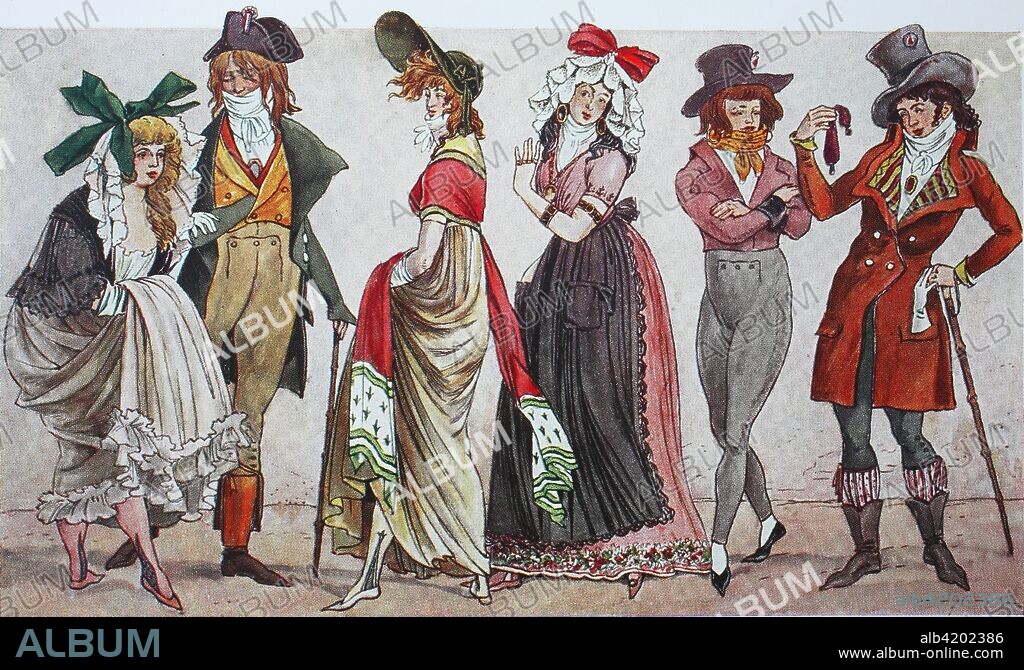This rectangular image, approximately 6 inches wide and 3 inches high, appears as an old cartoonish album card featuring six individuals—five women and one man—dressed in elaborate period costumes reminiscent of early 1800s British fashion. The background is light gray with a brown floor, and a thin light blue strip runs along the top. 

At the bottom edge of the card is a black footer. On its left side, in large blue letters, is the word "Album," while the right side bears the text "ALB4202386" in white, and underneath that, "www.album-online.com."

The figures are positioned as if on a stage, with the woman on the left walking arm-in-arm with the man towards the right, while the other women look on. The women wear corseted, floor-length dresses with aprons, both short-sleeve and long-sleeve varieties, embellished with bows, ribbons, and hats. Their hairstyles include bows and buns. Some women are dressed in breeches instead of dresses.

The man is adorned in breeches, an overcoat, and a captain's hat, with intricate elements like a high-collared shirt and ruffled sleeves. Footwear varies from pointed shoes, flat pointy shoes, to boots. Accessories such as canes and tall socks enhance their historical attire, as they stand and pose on the brown floor.